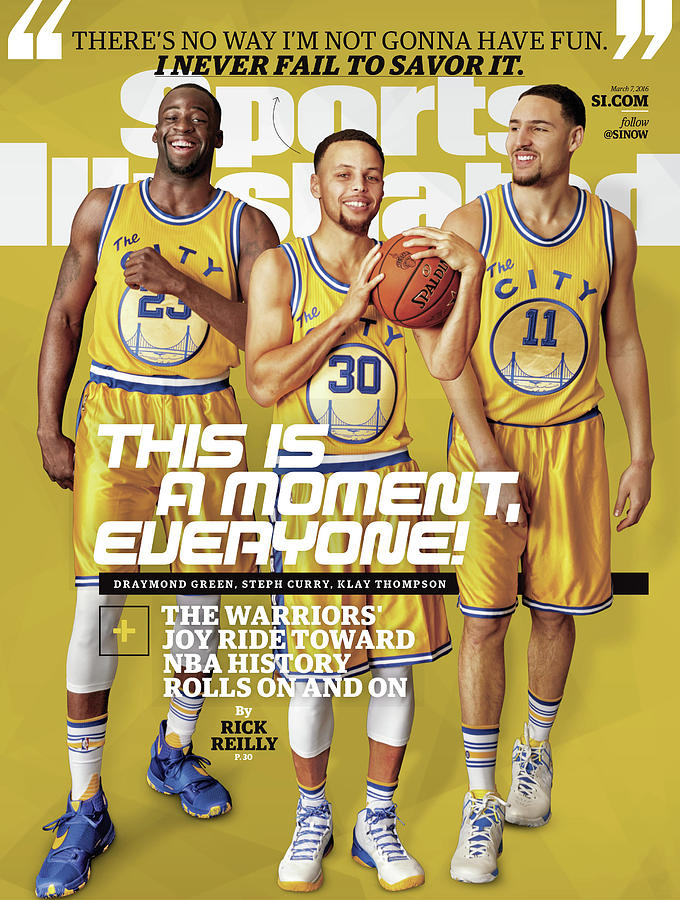This image is a vibrant Sports Illustrated magazine cover featuring three Golden State Warriors players: Draymond Green on the left, Stephen Curry in the center holding a basketball, and Klay Thompson on the right. The players are all dressed in the team's iconic blue and gold jerseys emblazoned with "The City," symbolizing Oakland. Above them, a motivational quote reads, "There's no way I'm not going to have fun. I never fail to savor it." In the center, bold text states, "This is a moment, everyone!" followed by the exclamation mark. Further text emphasizes the Warriors' exhilarating pursuit of NBA history, as outlined by Rick Riley. The trio is smiling against a striking gold background under the Sports Illustrated masthead, with Curry and Thompson in white and blue shoes, while Green sports blue shoes.